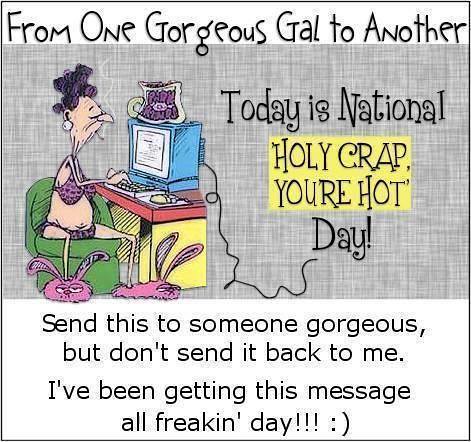This square image, outlined in black, has a comic book style and features a cartoon grandmother. At the top, set within a white rectangle with a handwriting-like font, it reads, "From one gorgeous gal to another." Below this, a wide, hand-markered gray rectangle spans the image. To the left, the cartoon grandma is seated in a green chair at a desk, wearing purple leopard print underwear (a bra and panties), pink bunny slippers, pearl earrings, and sporting messy purple and black hair. She is typing on a keyboard connected to a blue computer, with a mug on top of the monitor. On the right side of the image, in a yellow square, the text declares, "Today is National Holy Crap You're Hot Day." At the bottom, within another white rectangle, it says, "Send this to someone gorgeous, but don't send it back to me. I've been getting this message all freaking day!!!" followed by a smiley face.